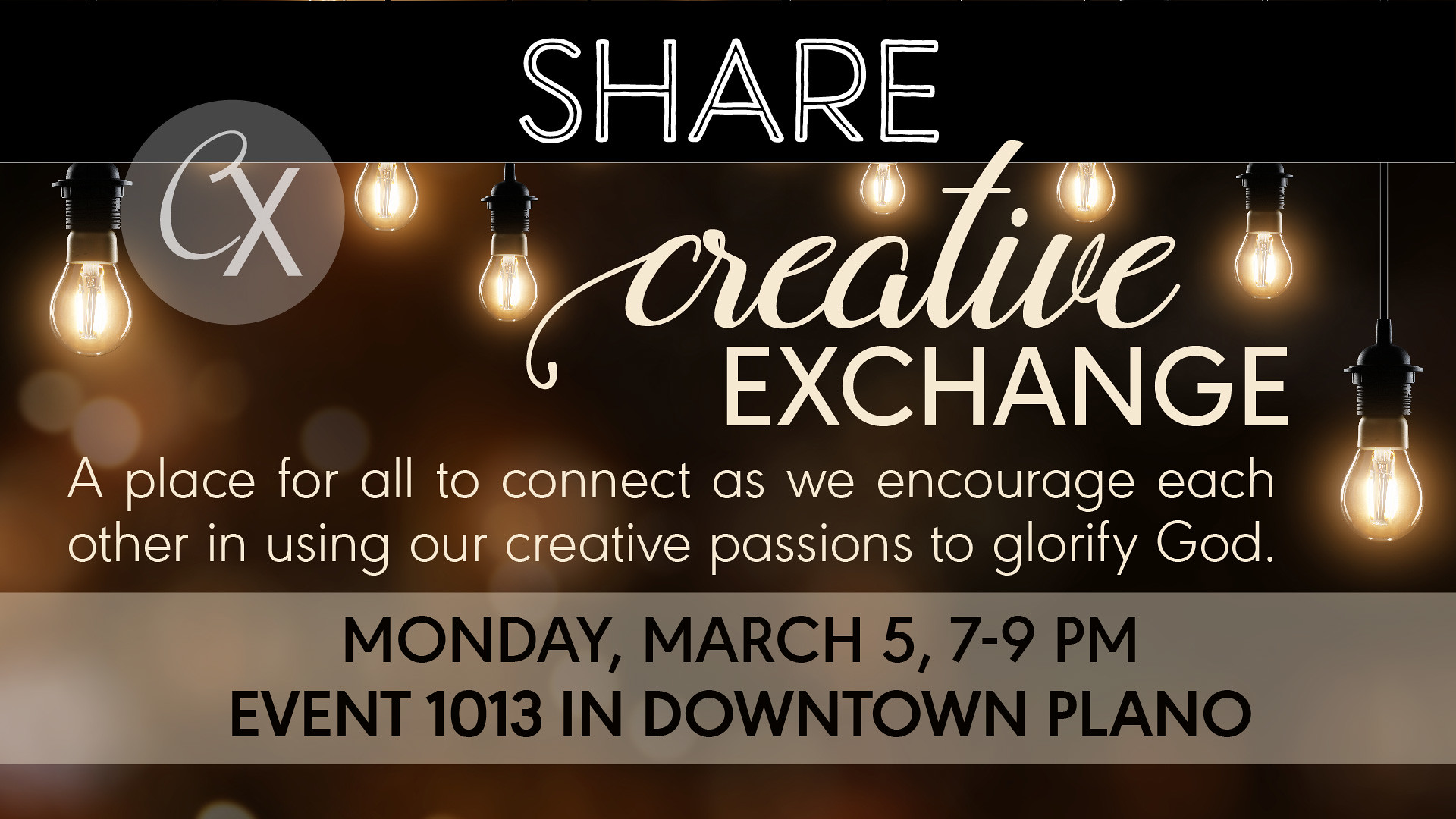The advertisement flyer for Creative Exchange features a black border at the top with the word "Share" written in bold white text. Below the border, the main image comprises a darker portion at the top, adorned with vintage-style hanging lights, casting a soft glow that creates subtle reflections in the background. Further down, the background transitions to a lighter and blurrier texture. Positioned at the upper left corner is a transparent circle containing the letters "CX" and the name "Creative Exchange." Beneath this logo, in clear white text, is the tagline: "A place for all to connect as we encourage each other in using our creative passions to glorify God." Additionally, a transparent white band across the bottom part of the flyer includes event details in black text: "Monday, March 5th, 7 to 9 p.m., Event 1013, downtown Plano."